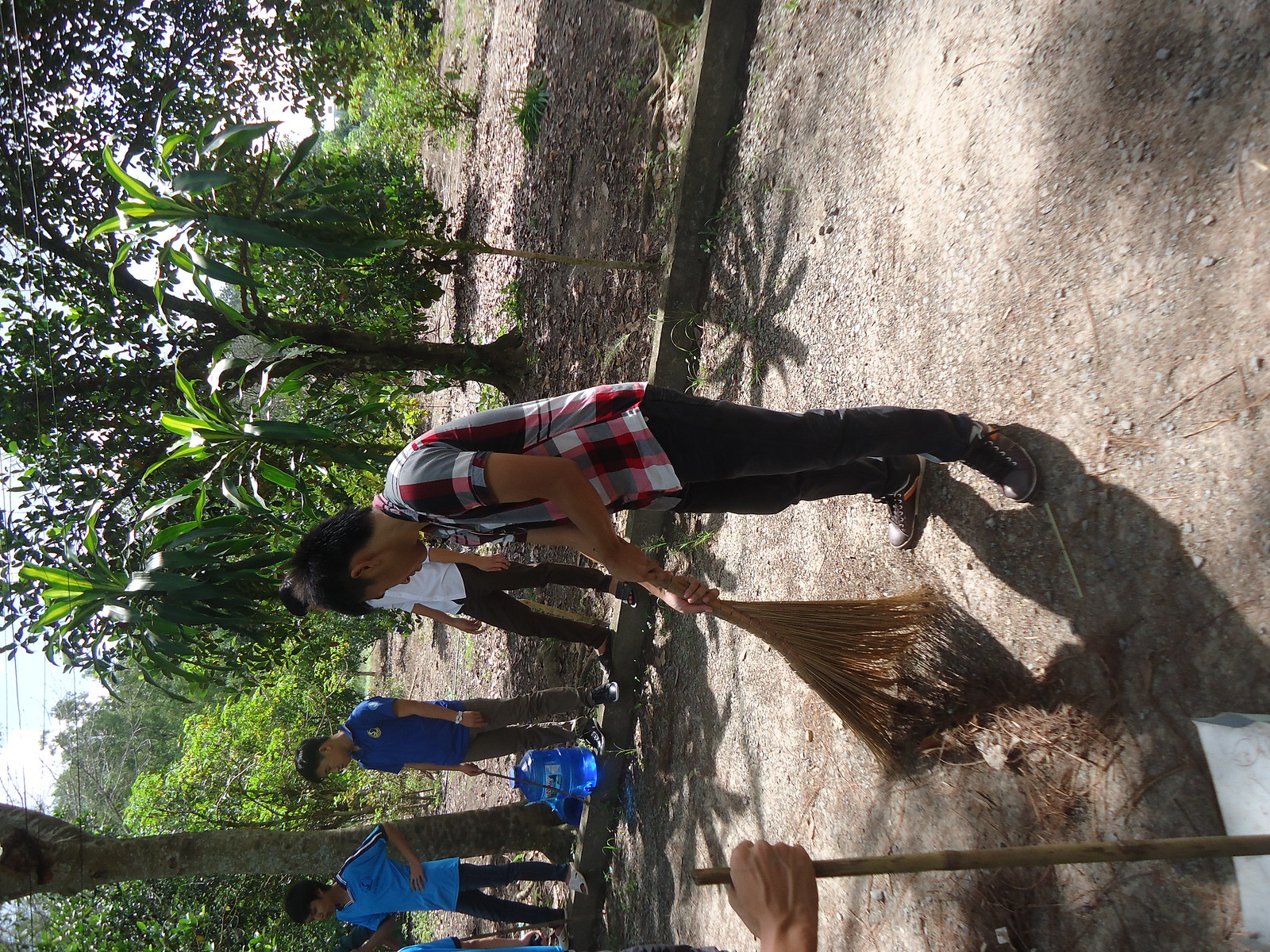The photograph, taken outdoors on a partly cloudy day, captures a scene set against a background of large trees with prominent palm leaves. The image is sideways and features four men. Three men are standing in a line on one side of a trench; the first man is wearing a blue jersey, the second man is in a blue T-shirt, and the third is dressed in a white shirt. The fourth man, positioned in the foreground, is grasping what appears to be a net. Also distinctive in the photo is a visible arm in the bottom corner, holding a long wooden stick, and another hand holding what looks like a dustpan. The ground beneath their feet is a mix of grass and dirt.